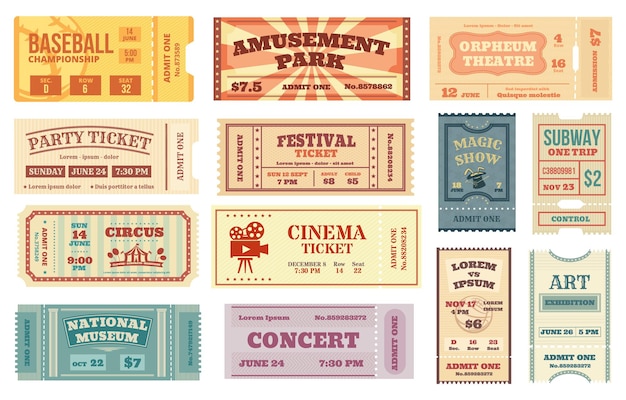The image is a meticulously arranged artwork showcasing a collection of admission tickets for various events. The tickets are laid out on a clean, white background and range in color and design, creating a visually appealing collage. In the upper left corner, notable tickets include ones for a Baseball Championship, Center Amusement Park, Orpheum Theater, Party, Festival, Magic Show, Subway One Trip, Circus, and Cinema. Additionally, there are tickets for the National Museum, a Concert titled "Lorem versus Ipsum," and an Art Exhibition. Most of the tickets feature a range of colors, predominantly in shades of pale beige with red or brown text, while a few stand out with brighter details: the Magic Show ticket has orange text on a green background, the Concert Ticket is rose-colored, and the National Museum ticket is a vibrant green. There are also two tickets that are primarily blue and one pink, adding to the diverse color palette. The varied and nostalgic nature of the small tear-off type tickets evokes a sense of vintage charm and curated artistry.